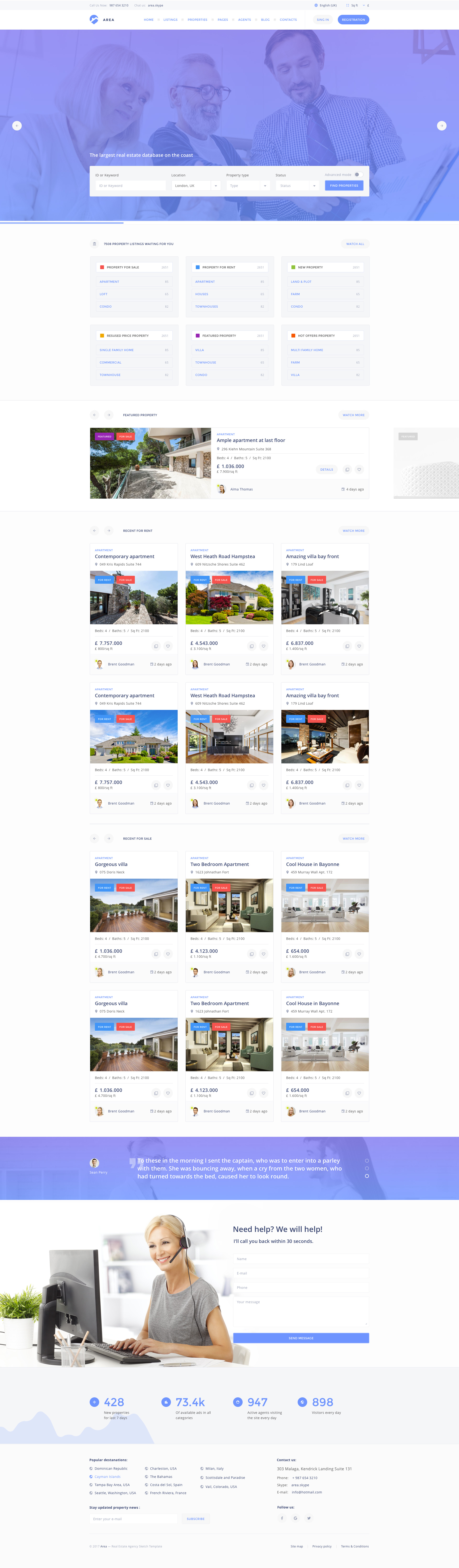This full-page screenshot captures a Realtor website with a clean, white background. At the top, a prominent blue header spans the width of the page. Centered within this header is a large rectangular navigation bar featuring drop-down menus for selecting area, price, bedrooms, and bathrooms, accompanied by a blue search button. 

Beneath this navigation bar are six small grey boxes, each containing different options for refining searches or accessing various features. These options lead to a comprehensive listing area, starting with a featured property prominently displayed. Below the featured listing, there are four rows of property thumbnails, with three listings per row. Each listing includes a detailed description above the property photo, and below, the price and additional property details are provided. The layout is meticulously organized, presenting each property in a neat square format.

At the bottom of the page, a large blue banner stretches across the site, underscoring the content. Directly under this banner, an image depicts a woman sitting behind a computer, wearing a headset, suggesting customer support or contact availability. To her left, there is blue text, although the screenshot's minimized state renders it unreadable, along with the webpage text. Despite the minimized view, the layout and visual elements, including property images, remain clearly distinguishable.